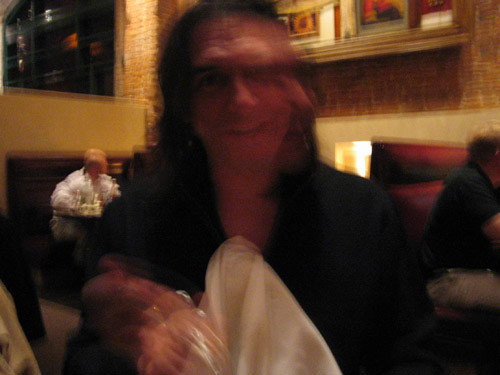The photograph is extremely blurry, capturing a scene inside a restaurant. In the foreground, there is a man with long hair wearing a black shirt, seemingly holding something indistinct that might be a white cloth or possibly his own blurred hand. Behind him, the restaurant's interior unfolds with a series of booths. One booth is partially visible with a person wearing a white, possibly fluffy, jacket, their gender indeterminable due to the blurriness. Above their head, there is an image of a building, and adjacent to it hangs a large picture featuring flowers. Below this picture, a lamp is placed on a table. To the right of this setup, another booth hosts a man with short hair, dressed in a black shirt and light-colored, possibly khaki, slacks. The general ambiance of the restaurant suggests a warm, adobe tan color palette on the walls. Overall, the double exposure and the extensive blurriness obscure many details, making the exact elements and scene challenging to discern.